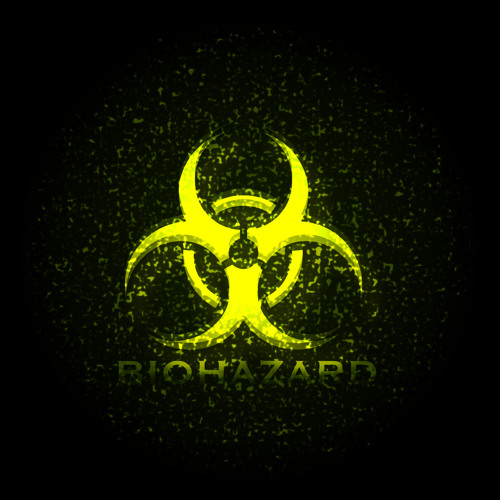The image is a simple square-shaped graphic with a black background featuring a stylized biohazard symbol in bright neon yellow. At the image's center is a distinct, captivating symbol comprised of three curved "petal-like" components resembling crescent moons, which are thick at their base and taper inward, yet they do not touch. These crescents are arranged in a manner that they connect at their thickest points, forming a central hole. Encircling these crescents is a neon yellow ring. Scattered throughout the background, there are tiny specks of neon yellow, akin to a star field or a dusting, adding a nuanced texture to the black space. At the bottom of the image, in faded neon yellow sans-serif all-caps font, is the word "BIOHAZARD." The text subtly blends into the background, contributing to the overall stark and cautionary visual effect of the image.